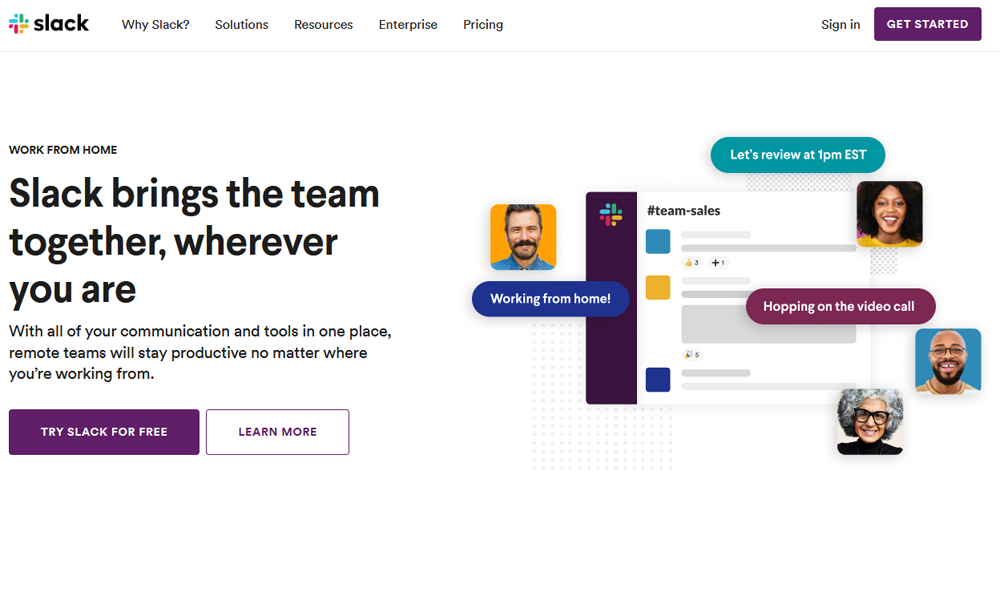The image showcases a webpage with a predominantly white background that appears to be the homepage for Slack, as indicated by the "Slack" logo prominently placed in the upper left corner. To the upper right, the navigation menu includes options like "Why Slack?", "Solutions", "Resources", "Enterprise", and "Pricing". Furthest to the right are two buttons: a "Sign In" button and a prominently featured purple "Get Started" button.

The main body of the page features a combination of descriptive text and imagery. On the left side, there's a section promoting remote work, with the text: "Slack brings the team together wherever you are. With all your communication and tools in one place, remote teams will stay productive no matter where you're working from." Below this, a purple button invites users to "Try Slack for Free," accompanied by a white "Learn More" button with purple text.

To the right, a picture depicts a communication chat window titled "team-sales," featuring four people—two women and two men, likely in their 30s or older. The chat includes comments such as "Let's review at 1 p.m. EST," "Working from home," and "Hopping on the video call." This visual aims to illustrate how Slack facilitates interaction within remote teams.

Overall, the webpage exhibits a clean and user-friendly interface, designed to showcase the capabilities and advantages of using Slack for team communication and collaboration.